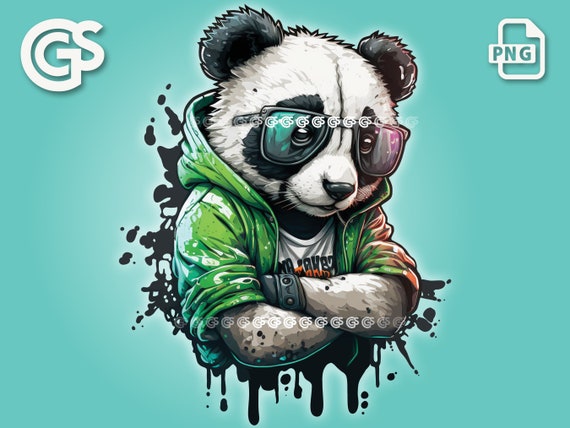This image is a detailed computer-generated illustration of a stylish panda. The panda is sporting a pair of sunglasses and is gazing off to the right, exuding a cool demeanor. He is dressed in a trendy green hoodie layered over a white shirt, which has some writing partially obscured by his crossed arms. The panda also appears to be wearing gloves, and there are distinct white spots on the right sleeve of his hoodie. On his left sleeve, a subtle red glow adds an intriguing visual element to his appearance. The background features a dark, inky texture with scattered watermarks, including a prominent design on the top left resembling a "C" or "G" intertwined with a "C" and an "S" beside it. Additionally, there is a small graphic design icon on the top right depicting a paper with "PNG" written on it. The overall scene is set against a gradient backdrop blending green and blue hues.